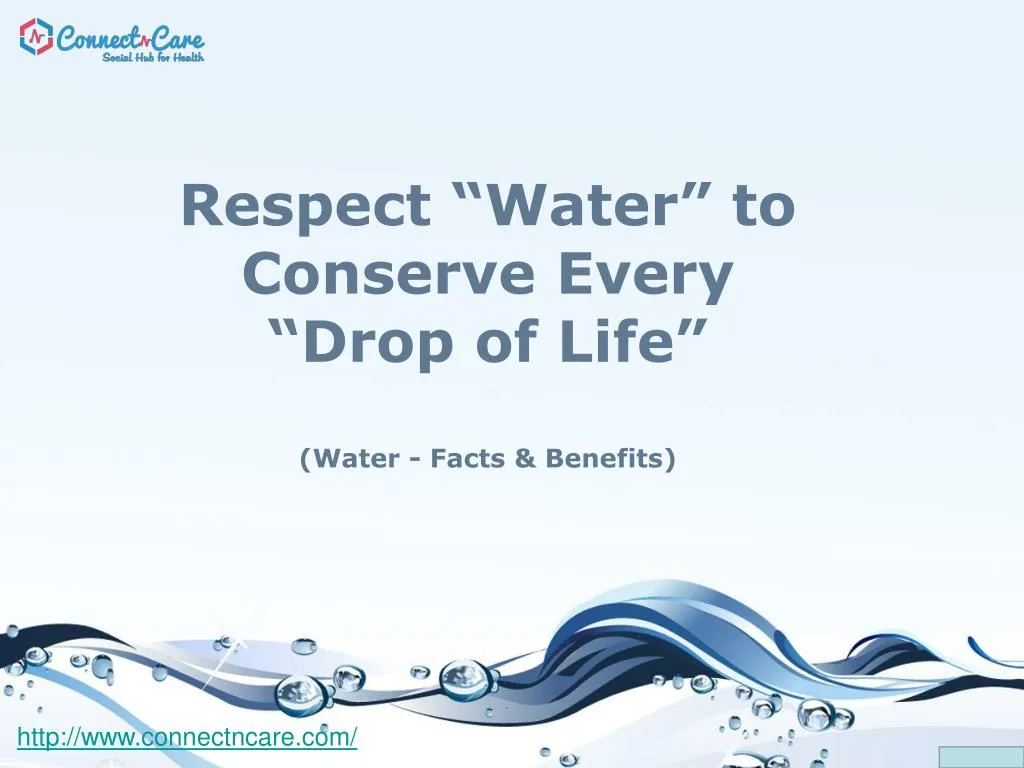The poster emphasizes the importance of water with a detailed and visually appealing design. The background starts with a light blue color at the top, transitioning to white at the bottom. In the top left corner, there is a hexagon-shaped logo with red and green lines along the edges, featuring the letter "N" inside. Next to the logo, the text "Connect and Care, social help for health" is displayed.

Prominently in the center of the poster, the message "Respect water to conserve every drop of life" is written. Beneath this inspiring message, the text reads "Water - Facts and Benefits." At the bottom of the poster, a stream of water flows horizontally, accompanied by bubbles in different sizes and shades of blue, enhancing the elemental theme. Additionally, a blue curvy line and ribbon-like waves run across the bottom, adding to the fluidity of the design. The bottom left corner includes a link to the website, "http://www.connectandcare.com," providing further information.